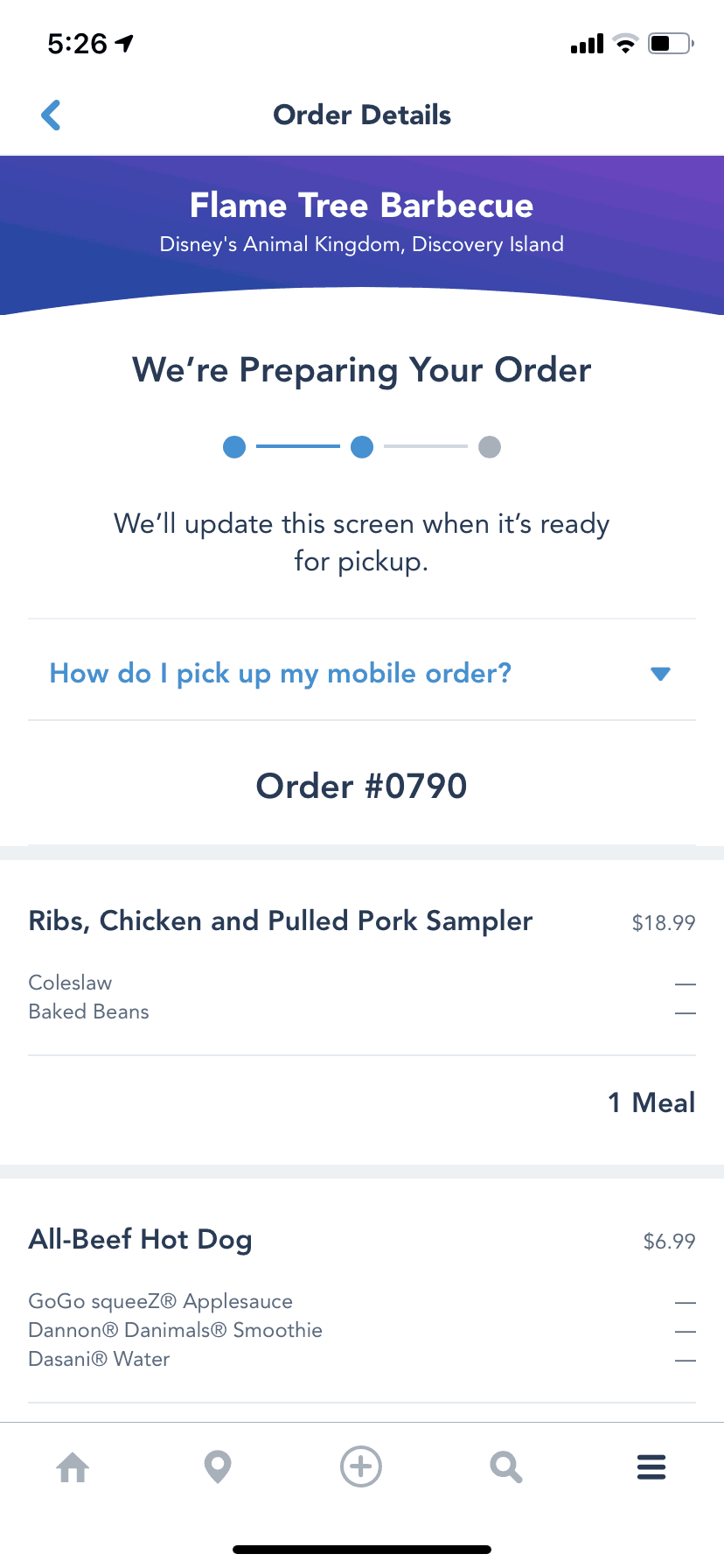**Detailed Caption:**

This image is a screenshot of an order confirmation page from either an app or a website. At the top, there is a white section displaying "Order Details," accompanied by a blue back arrow on the left side. Beneath this is a distinct blue header with a uniquely curved bottom edge that arches upward. In this blue section, the establishment name is presented in white text: "Flame Tree Barbecue, Disney's Animal Kingdom, Discovery Island."

Directly below the blue header, the status of the order is communicated with the message "We're preparing your order." This is visually reinforced with a progress bar comprising three steps represented by circles and lines. The first circle, the first connecting line, and the second circle are all highlighted in blue, indicating progress. The section also mentions that the screen will be updated once the order is ready for pickup. 

Further below, a clickable blue text option reads "How do I pick up my mobile order?" accompanied by a drop-down arrow on the right. Lastly, the order number "0790" is displayed for reference.